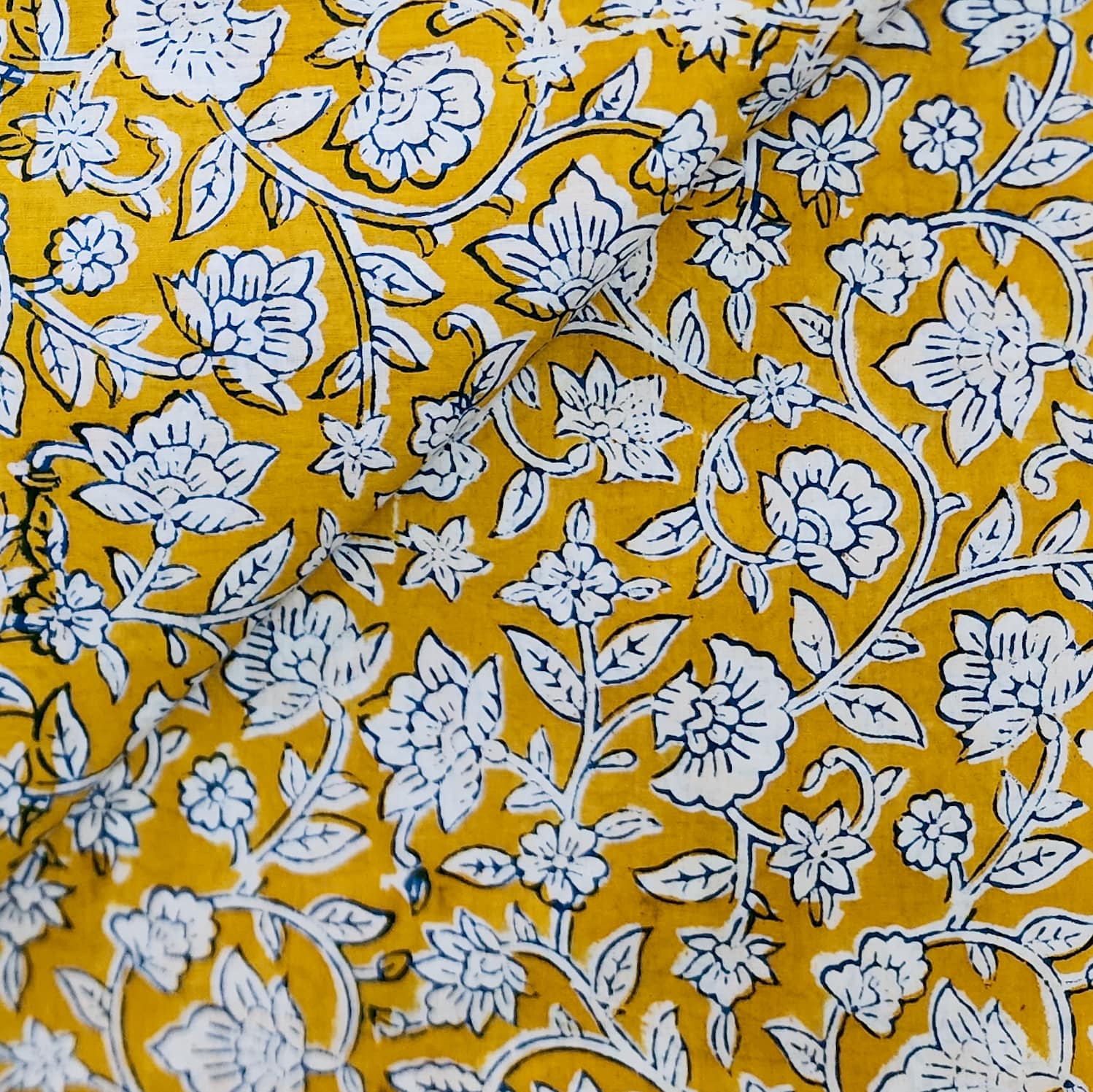This close-up photograph captures the intricate design of a dinner tablecloth with a rich yellow mustard-colored background. The tablecloth features an elegant, all-over floral pattern primarily rendered in black and white. The flowers, some budding with three to six petals and various sizes, are outlined meticulously in black ink with delicate, black lines accentuating the petals. They are intertwined with winding vines and stems, which also bear leaves detailed with fine, black vein lines. These twisty vines and floral motifs extend across the entire fabric, covering it from corner to corner. The tablecloth appears to be slightly creased, accentuating its fabric texture. Notably, there are minor printing imperfections where the colors seem slightly misaligned, reminiscent of a lithograph printing method. The overall effect is one of a vibrant, detailed, and organic floral design against a warm yellow backdrop, creating a visually rich and textured tablecloth.